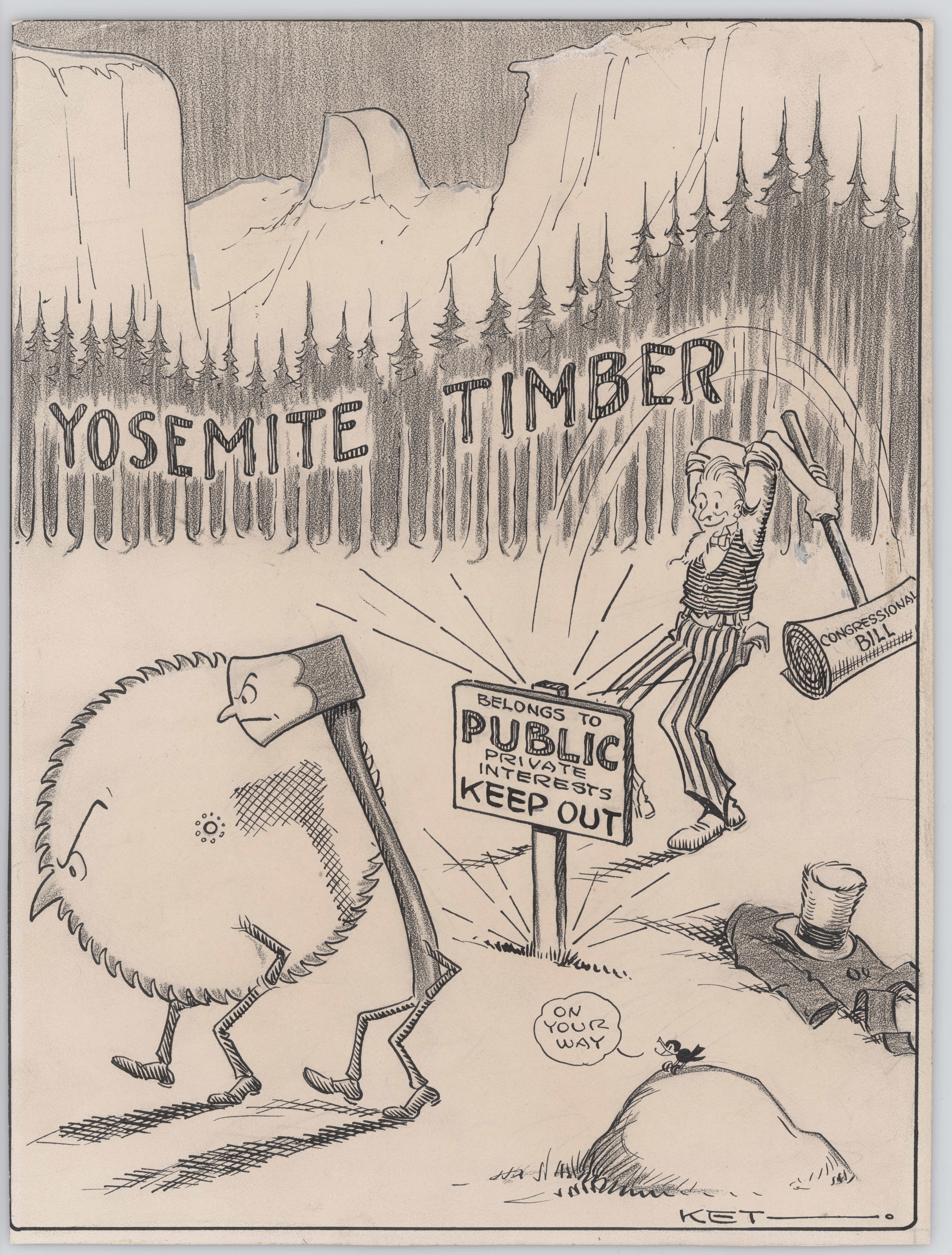This vertically aligned, black-and-white sketched cartoon, likely a newspaper clipping, captures a satirical scene. At the top, it depicts detailed vertical lines representing pine trees with pointed tips, set against a sketched mountainside. Above the mountains, a solid, pencil-shaded sky serves as the backdrop for the bold, all-caps text "YOSEMITE TIMBER." Below this, the bottom half of the image focuses on an older man with a long beard, identified as Uncle Sam. He wears striped pants and a matching shirt, and holds a massive mallet labeled "CONGRESSIONAL BILL" poised behind his head. Uncle Sam is preparing to hammer a sign into the ground. The sign reads "BELONGS TO PUBLIC PRIVATE INTEREST KEEP OUT." To the side, two anthropomorphic characters—a thin, Gumby-like figure with a rectangular face, and a brown, poofy bird—both sporting expressions of anger and disappointment are seen walking away. The scene encapsulates the tension between public and private interests in environmental conservation efforts.